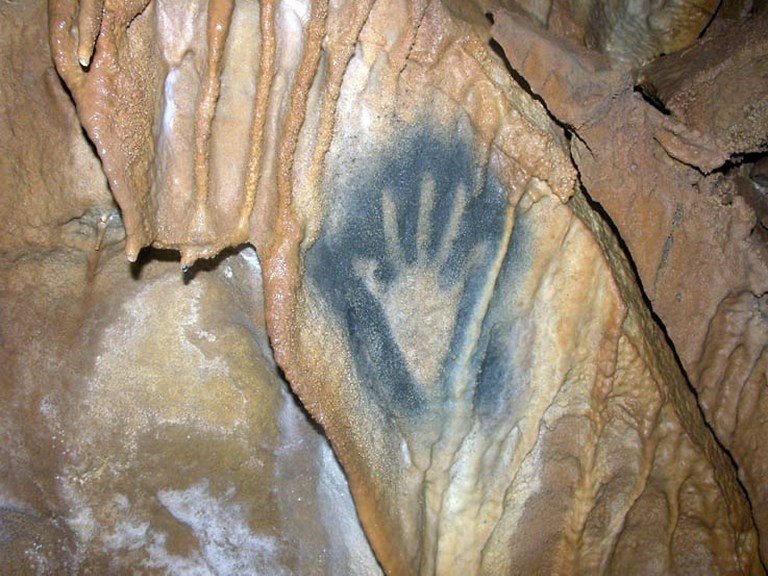The image is a large square close-up of an intricately detailed cave wall, bathed in artificial light that illuminates its textured nuances. Predominantly composed of various shades of brown, the central focus is a light brown handprint surrounded by a halo of black spray paint, giving the impression that the hand was once pressed against the rock. There are vertical streaks descending from the upper left to the lower right. Below these streaks, on the left side, a secondary rock formation displays a blend of brown, light brown, and white hues, potentially due to natural mineral deposits. A noticeable crack stretches from the lower right corner upward, intersecting the image, and another crack meanders from the lower center toward the left upper portion. To the right, a darker brown rock face captures the eye with its weathered, almost smooth appearance, while at the top, mineral deposits resemble solidified drip marks. The lower left area showcases more brown rock embellished with natural white formations, suggesting mineral presence. Visual elements include vertical lines and zigzag patterns etched into the rock's surface, adding to the complex texture and natural beauty of the scene.